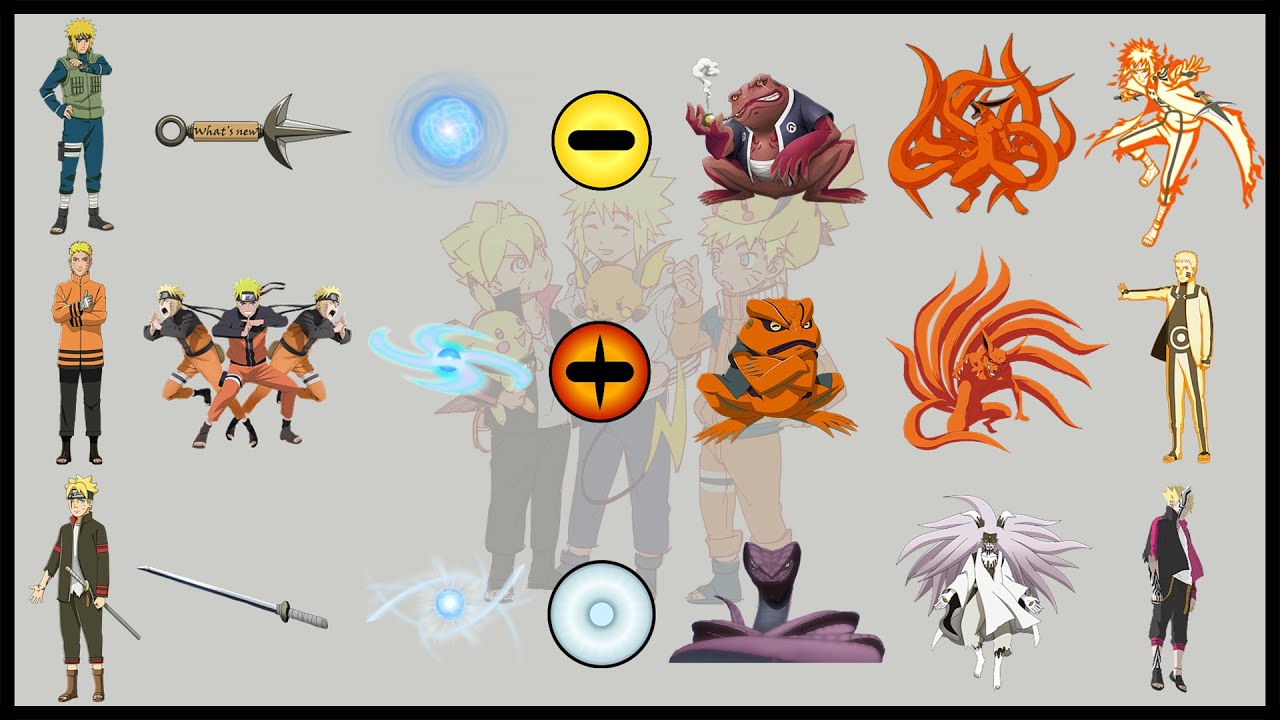The image features a detailed and highly colorful scene set against a gray background. In the faded center, there are three cartoon children with blonde hair, while the left side showcases three male figures stacked one on top of another. The top figure has blonde hair and appears to be wearing an army suit, wielding a pointy weapon resembling a knife. Directly below him, another blonde figure in an orange jacket is shown in three different action poses, emphasizing movement. The third figure, at the bottom, is a blonde man dressed in a green and red military outfit, brandishing an elongated sword.

The overall composition includes a myriad of animated objects and characters portrayed in an anime or cartoon style. Colorful elements such as angry frogs, a maroon crouching frog, and a uniquely designed orange frog with its arms crossed add to the visual interest. Additionally, a fox-like creature with multiple tails or legs—reminiscent of an octopus—makes this image even more captivating.

There are three colored circular shapes positioned centrally: yellow at the top, orange in the middle, and light blue at the bottom, each accompanied by nebulous, space-like figures. The array of characters and symbols scattered throughout the image presents a vibrant tapestry dominated by shades of black, gray, yellow, brown, orange, blue, purple, and light purple. The scene also includes a serpent and various mutants, contributing to the complexity and dynamic nature of the illustration.

Overall, the image appears to be heavily influenced by Japanese anime, with echoes of Dragon Ball Z–style characters, and leaves an impression of an intricate, well-positioned collage filled with lively and assorted elements.